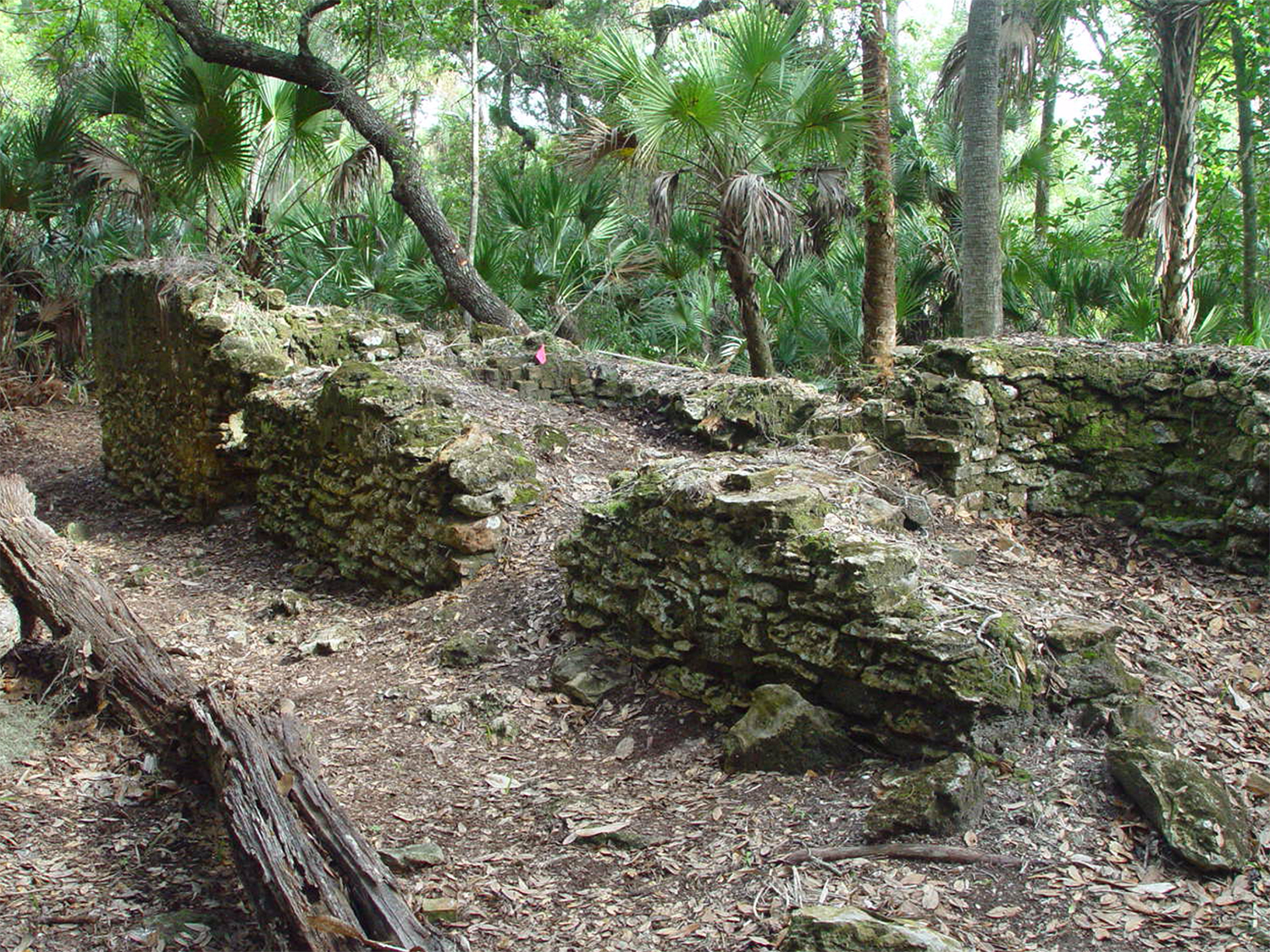This photograph captures the ruins of an old structure, possibly a house or a barn, situated in a dense, tropical forest abundant with palm trees and some birch trees. The remaining stone walls of the building are uneven and covered in green moss and algae, indicating their age and abandonment. In the foreground, there are several fallen, rotting logs, and on the left side, decayed tree stumps add to the scene of neglect. The ground is a mixture of gray dirt, rotting and decaying leaves, devoid of any grass. The forest seems to envelop the ruins, with the healthy palm trees showcasing brown trunks and vibrant green fronds stretching as far as the eye can see. Amidst the greenery, there is a small, vague patch of pink near one corner, possibly a piece of trash like a deflated balloon. Part of the ground next to the ruins appears to be a walking trail. Through small clearings in the dense foliage, glimpses of the sky are visible, adding light to the otherwise overgrown and wild setting.